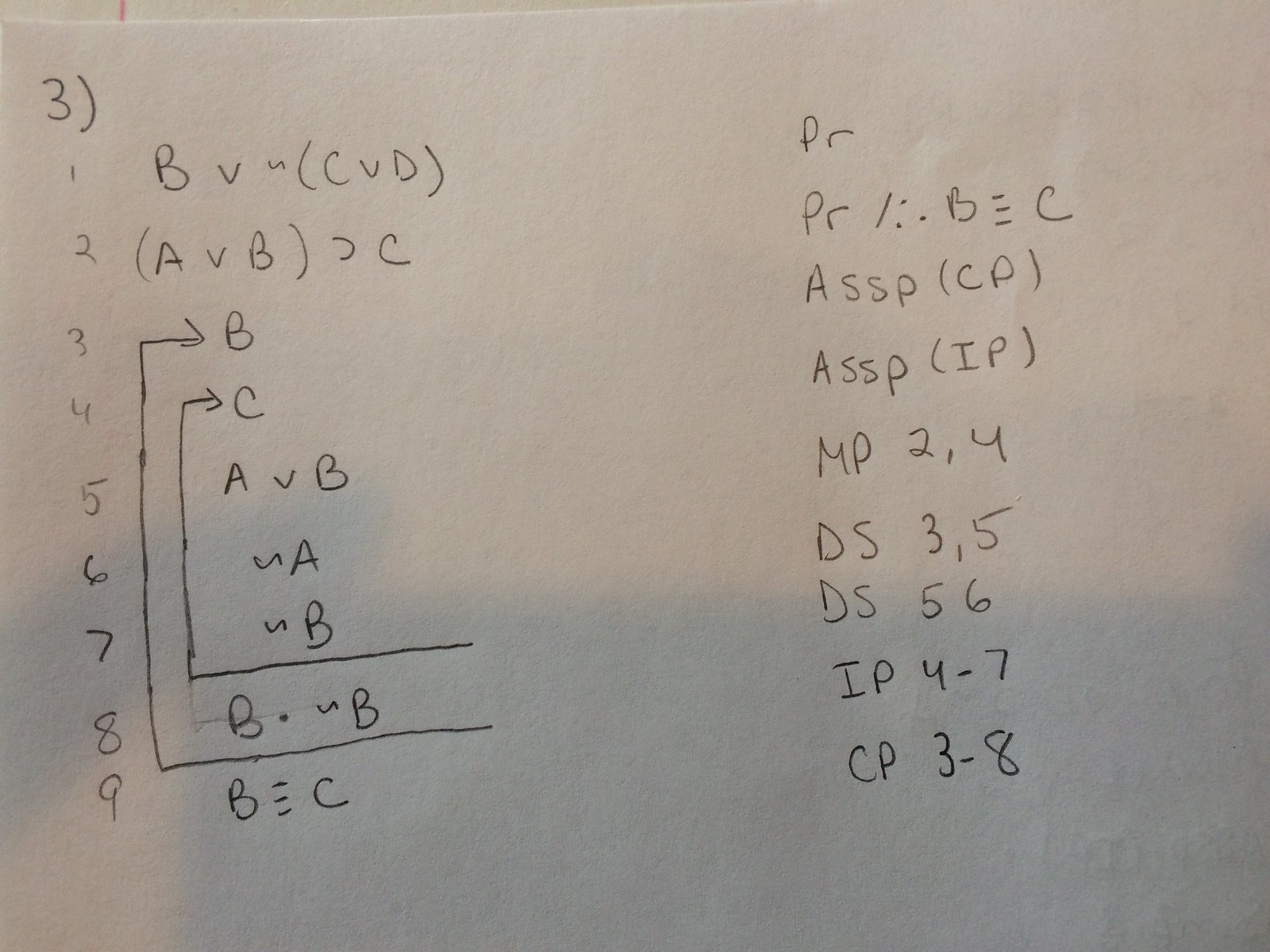This image features a page covered with intricate mathematical formulas that could potentially be interpreted as crib notes for a test or codes representing various symbols. In the upper left-hand corner, a prominent number "3" is visible. Below the "3," there is a vertical column of numbers ranging from one to nine, each paired with clusters of letters. For instance, in the number one position, the letters "BV" and "CVD" appear. 

On the right-hand side of the page, there is another column filled predominantly with letters such as "P," "R," "A," "S," "S," "P," "M," "P," and "D," with some of these letters repeating frequently. Meanwhile, the left-hand side is marked by numerous appearances of the letters "A," "B," "C," and "D." 

The page is divided into two distinct sections, with the number "3" seeming to delineate the left column, and "PR" marking the separation for the right column. Both columns are densely packed with repeated formulas and letter combinations, making it challenging to decipher the exact purpose or contents of the page.